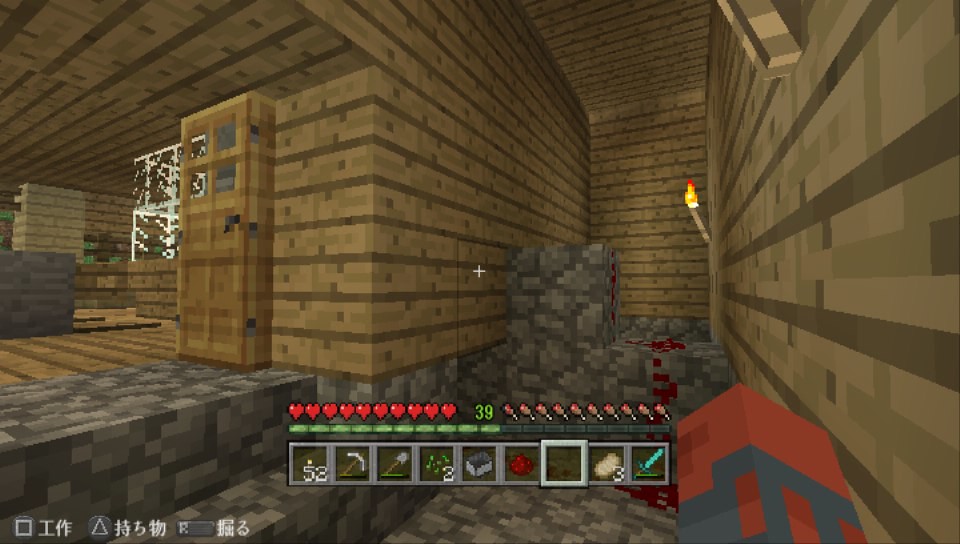This image is a screenshot from the video game Minecraft, recognizable by its distinctive blocky graphics. The image is roughly 50% wider than it is taller, presenting a first-person view of the player's perspective. The scene appears to be set inside a constructed building with stone floors and wooden walls featuring horizontal brown stripes. 

At the bottom of the screen, detailed player information is visible, indicating full health represented by multiple hearts and hunger bars showing meat legs. The number 39 in green signifies the player's level. The player's inventory is displayed, showing 9 items including a torch (with a quantity of 53), a pickaxe, a shovel, seeds, a metal box, red material, three potatoes, and a diamond sword. To the right, a fist with a red sleeve and a gray wrist can be seen, likely the player's in-game avatar.

On the left side of the hallway, a wooden door and stone stairs lead up to another room, which also appears to be constructed of wood. Further in the distance, glass panes are visible. A torch mounted on the wooden wall provides light, and a notable red block with black features lies in the foreground, possibly representing some in-game item or material. Some gray blocks are positioned on the far side of the room, which also contains what appears to be red blood-like material. White Japanese text and controller directions (a square and a circle) are located in the lower left corner, adding to the immersive game interface.